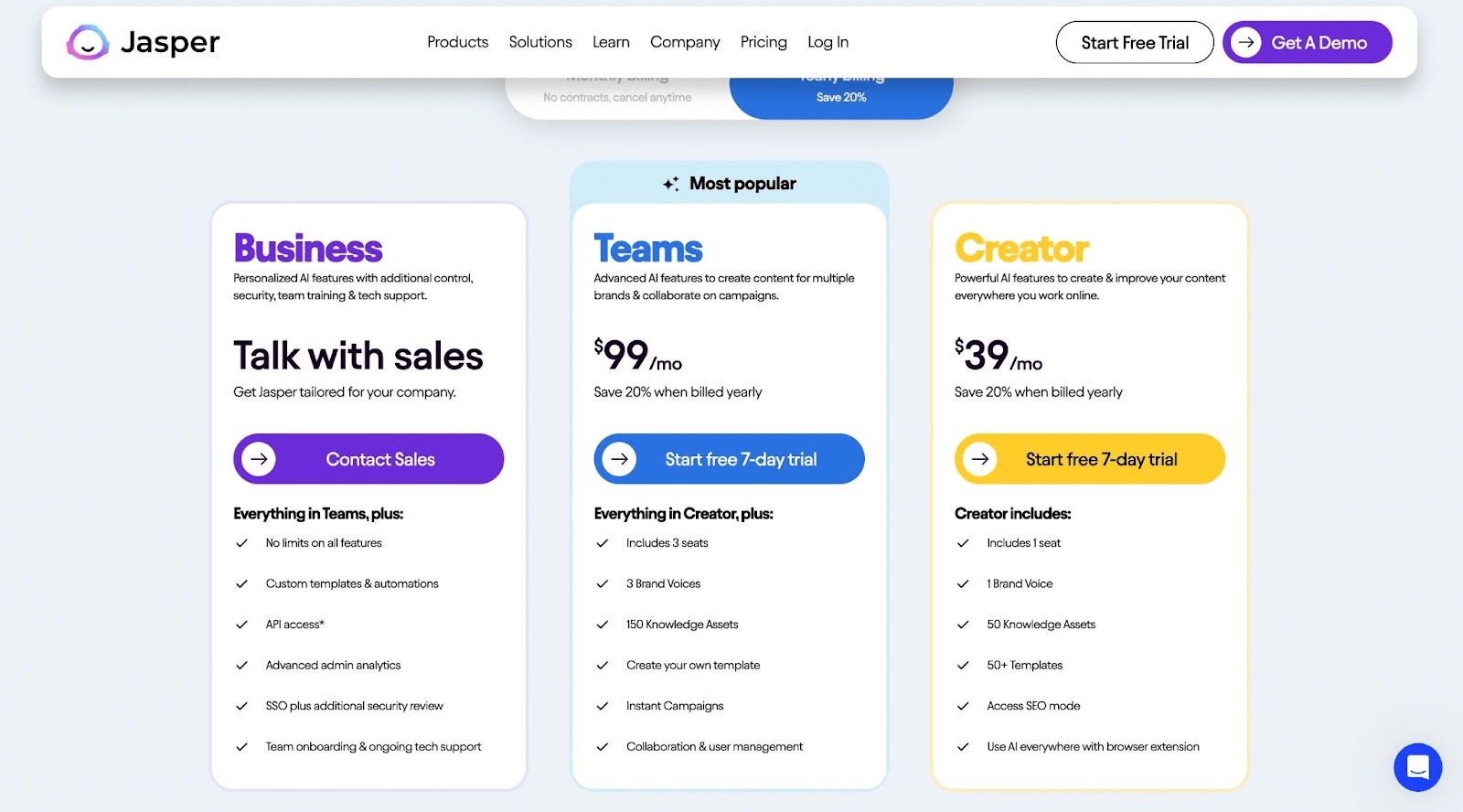**Detailed Caption for Jasper AI Pricing Plan Page:**

The Jasper AI Pricing Plan page is meticulously designed to offer clear and comprehensive details about the different subscription plans available. Each plan is distinctively color-coded for easy differentiation and is tailored to meet various needs, from individual creators to large businesses. 

- **Business Plan:** This option is designed for enterprises requiring personalized AI features with advanced control, security, and support. It includes comprehensive offerings such as custom templates, animations, API access, advanced admin analytics, team training, tech support, and team onboarding. Pricing is customized based on specific company needs, and interested users are encouraged to contact sales for a tailored solution. This plan encompasses all features from the Teams plan without any limits, ensuring robust and scalable AI-driven tools for large organizations.

- **Teams Plan:** Priced at $99 per month with a 20% discount for annual billing, this plan is perfect for teams working on multiple brands and collaborative campaigns. It includes advanced AI features along with support for three seats and three brand voices. Users benefit from 150 knowledge assets, the ability to create custom templates, launch instant campaigns, and manage collaboration effectively. A seven-day free trial is available for users to experience the plan before committing.

- **Creator Plan:** For individual creators or small teams, this plan provides powerful AI capabilities for content creation and improvement across various online platforms at $39 per month. The plan includes one seat, one brand voice, and 50 knowledge assets along with 50 templates. Users also gain access to SEO mode and a browser extension that integrates AI tools seamlessly into their workflow. A seven-day free trial allows users to test the features before subscribing.

At the bottom of the Teams and Creator columns, a footer section invites users to explore trending playlists, enhancing the user experience. The clean and visually appealing layout guides visitors effortlessly through the distinct features of each pricing plan, simplifying the decision-making process for potential Jasper AI subscribers.